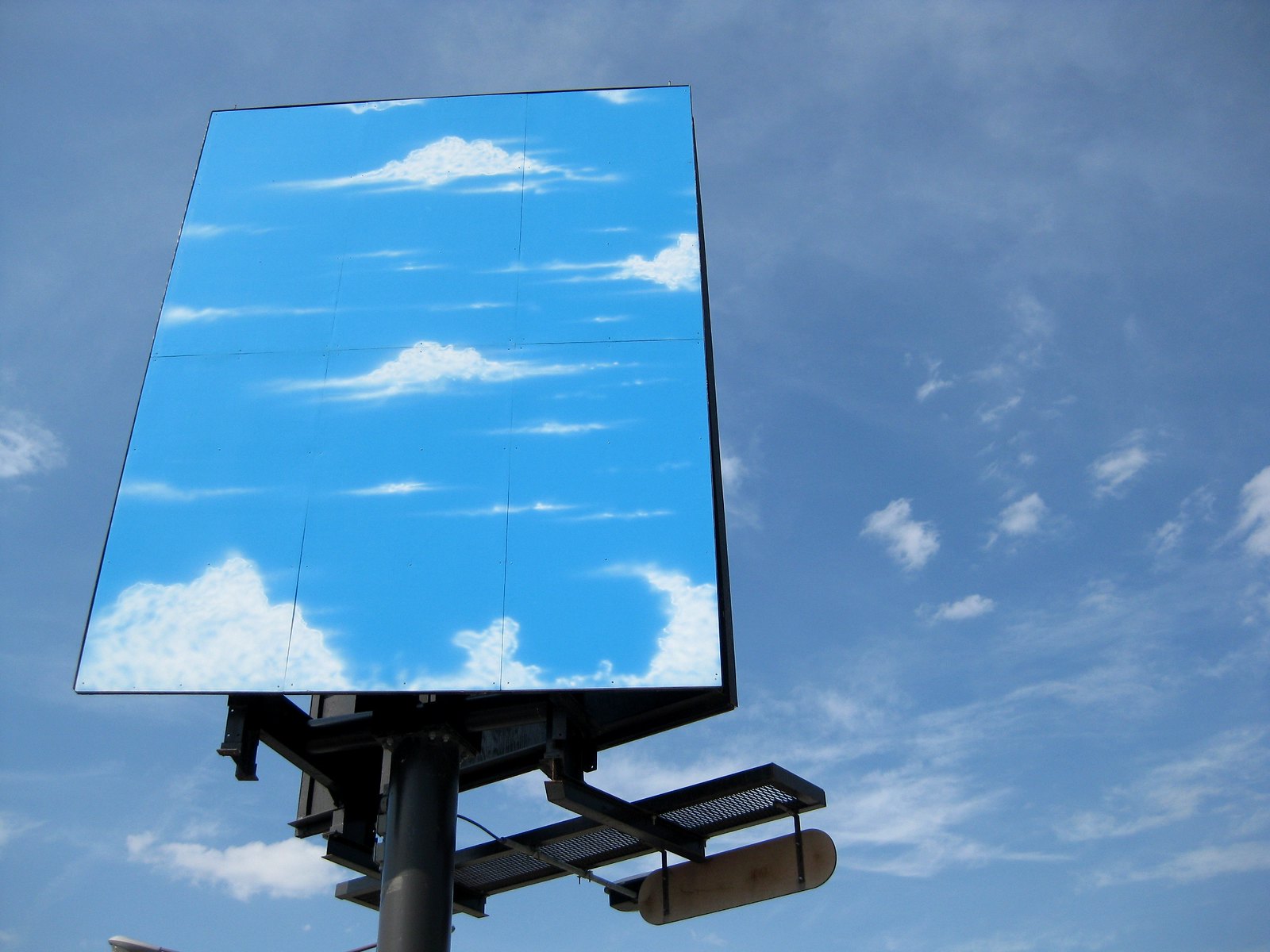The photograph captures a large, double-sided metal billboard towering over a main motorway. A sturdy platform is positioned at its base, designed to provide a workspace for individuals tasked with updating the advertisements on the billboard. Suspended beneath the platform is a rectangular sign, resembling the shape of a skateboard with rounded edges, which likely displays the name or logo of the company responsible for the billboard.

Additionally, an overhead spotlight is mounted under the platform, intended to illuminate the billboard during nighttime, ensuring visibility for motorists. On the bottom left of the image, a streetlamp is partially visible, further emphasizing that the billboard is located alongside a significant roadway.

Currently, the billboard displays sections of a vibrant blue sky with scattered white clouds, contrasting sharply with the actual sky in the background, which presents a more subdued lilac-mauve hue. The difference in sky tones between the billboard image and the natural horizon creates an intriguing visual contrast.